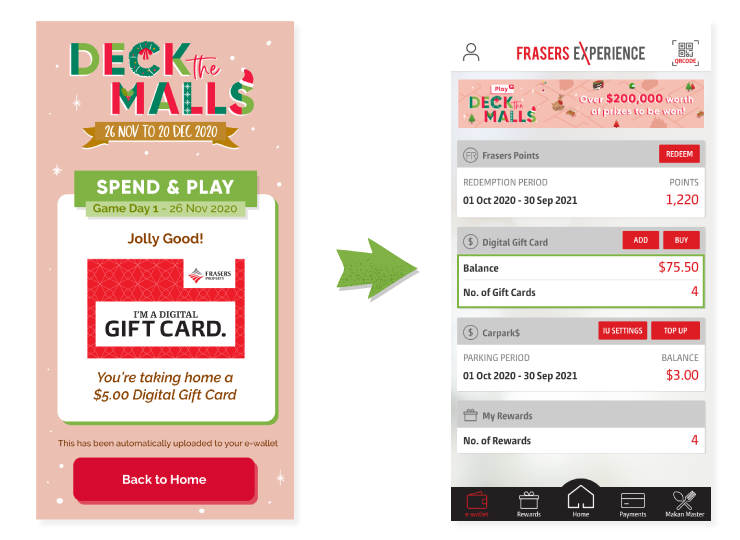This image showcases the interface of a mobile app, possibly named "Fraser's Experience" or "Deck the Malls," displayed on a smartphone screen. The app appears to be promoting a holiday-themed event or game called "Deck the Malls," which runs through December 2020.

On the left side of the screen, an image features the event title "Deck the Malls," with a green arrow pointing towards the right side of the interface. Below the title, there is a vibrant green button labeled "Spend and Play, Game Day 1." Further down, the section shows a red digital gift card on a white background, celebrating the user with the message, "Jolly Good! You're taking home a $5 digital gift card." At the bottom of this image, a red button prompts navigation with the text "Back to Home."

On the right side of the screen, the app section branded "Fraser Experience" is visible. This side mirrors the left with a similar small rectangular overlay. Below this, another rectangular segment displays the option to "Redeem" points, indicating the user has accumulated 1,220 points in red font. Further down, the app tabulates the user's "Digital Gift Card Balance" as 7550 in red, and tracks "Number of Gift Cards," listing a total of 4. Further options listed below include "Car Park" and "My Rewards." Within a white rectangle, the app highlights the "Number of Rewards" which is also 4.